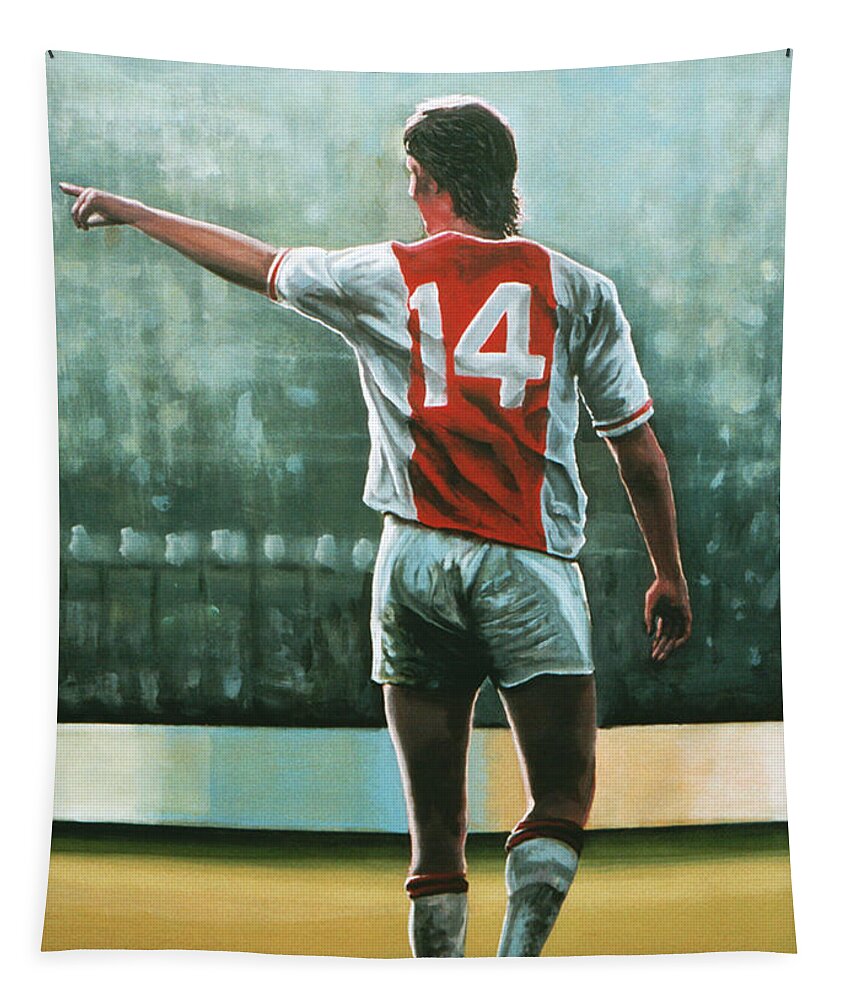This is a color image depicting a tapestry featuring a detailed painting of a soccer player. The player is viewed from behind, turning his head to the left while pointing his left arm upward, appearing to gesture toward the audience. He has dark hair and wears a white jersey with a prominent vertical red band down the middle, housing the number 14. His uniform includes white short shorts and knee-high white socks with red banding at the top, suggestive of shin pads beneath. The background is an abstract, impressionistic blur, resembling a crowd of fans in a stadium, though it is murky and indistinct. The tapestry itself is secured by two push pins at the top, and the scene unfolds on what looks like dirt ground within an arena. The overall artwork is taller than it is wide, adding a dynamic vertical emphasis to the composition.